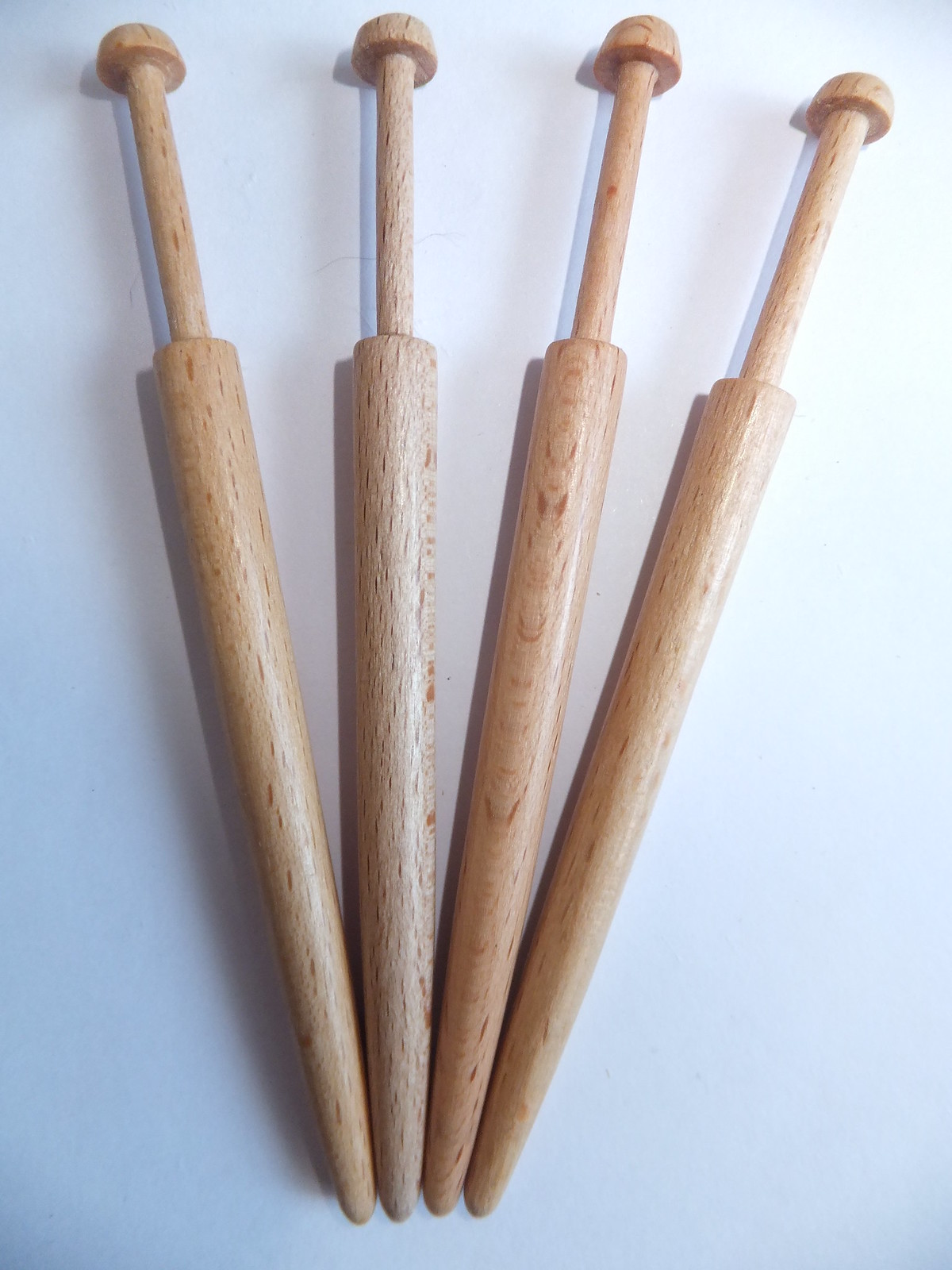The image displays four wooden objects resembling darts, each set against a white background. These objects are crafted from brown wood and display noticeable marks and minor cuts. They feature small rounded points at their tips which converge closely together, fanning out slightly as they extend upwards. The objects gradually widen from the tips into a broader base and then taper into slender, handle-like shafts. Each handle is capped with a small dome shape. The light source positioned behind the camera casts soft shadows onto the surface, revealing the textured details of the wood.